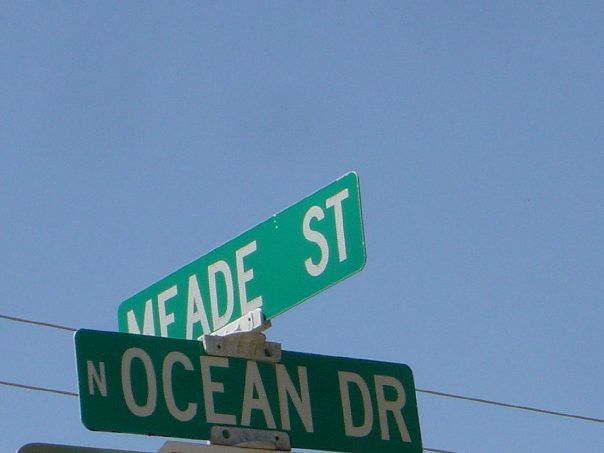In this horizontal rectangular outdoor photograph, taken in bright daylight against a clear blue sky, the focus is on two intersecting street signs mounted at the top of an unseen pole. The green signs with bold white capital lettering stand out prominently. The lower sign, slightly obscured by utility wires that cut diagonally across the bottom right, reads "N OCEAN DR," with the smaller 'N' for North and 'OCEAN DR' in larger, bold letters. This sign is secured by metal brackets on the top and bottom. Perpendicular to it, the upper sign reads "MEADE ST," although the 'M' is partially obscured by the sign below. Both signs are typical American rectangular street signs, easily identifiable and clearly mounted with bolts on a steel structure. The crisp, blue sky background with visible power lines completes the scene, adding a touch of urban infrastructure to this sunny day photograph.